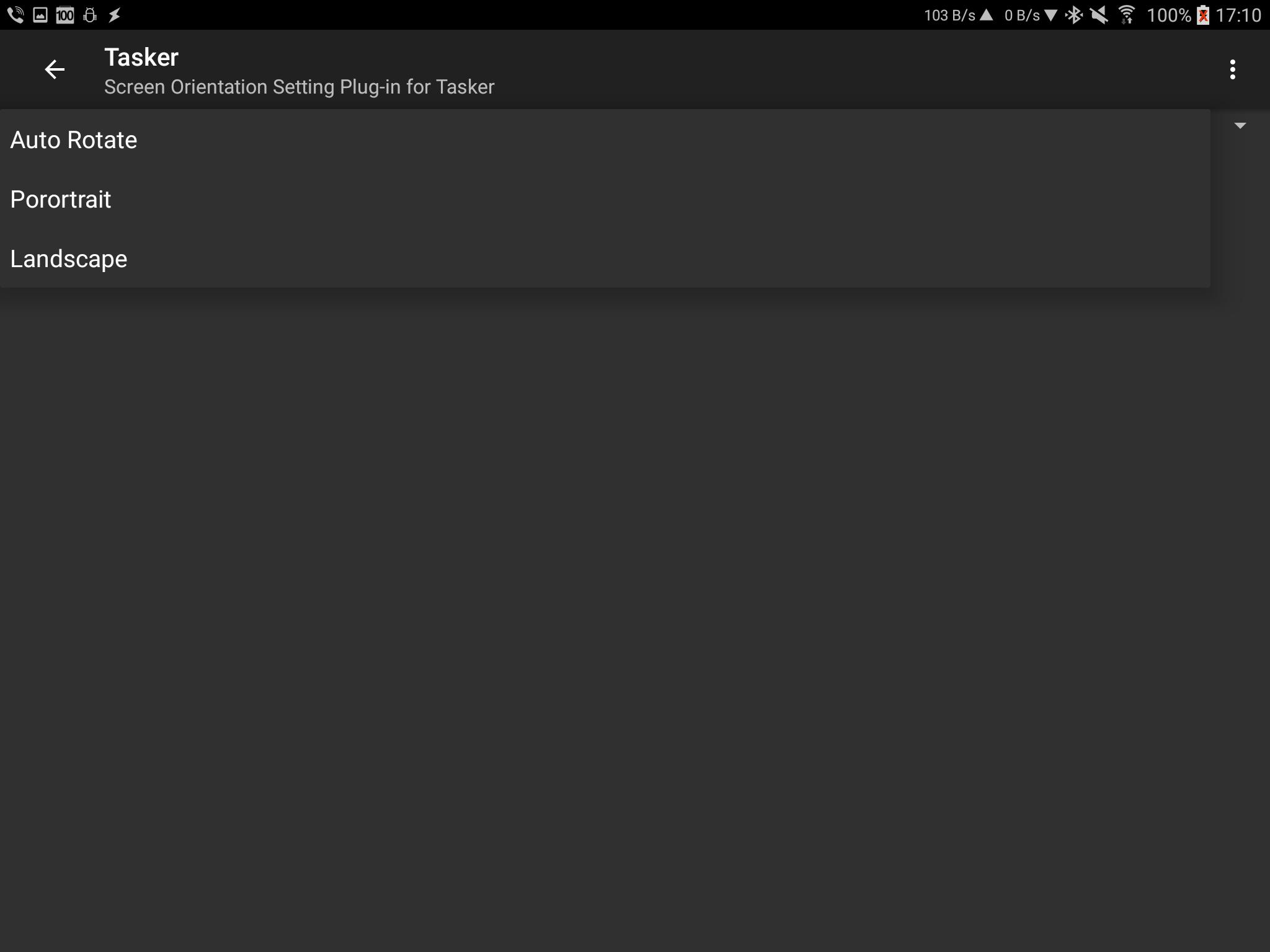The image is a screenshot from a smartphone displaying various status icons and information. In the top left corner, there is a handset icon followed by an unrecognized icon, a "100" indicator, another unrecognized icon, and a lightning bolt symbol. The top right corner shows a "103 B/s" label next to an upward-pointing triangle, a "0 B/s" label next to a downward-pointing triangle, a Bluetooth icon, an unrecognized icon, a Wi-Fi icon, and a fully charged battery icon at 100%. The time is displayed as 17:10.

Beneath the status bar, on the left side, an arrow points left with the text "Tasker - Screen Orientation Setting Plug-in for Tasker". On the far right, there is a vertical ellipsis icon and another downward-pointing triangle. Below this, the text "Auto Rotate" is visible, followed by "Pull Roll Trick", and then "Landscape". The lower portion of the image is a darker shade, containing no additional elements or text, making it an empty space.